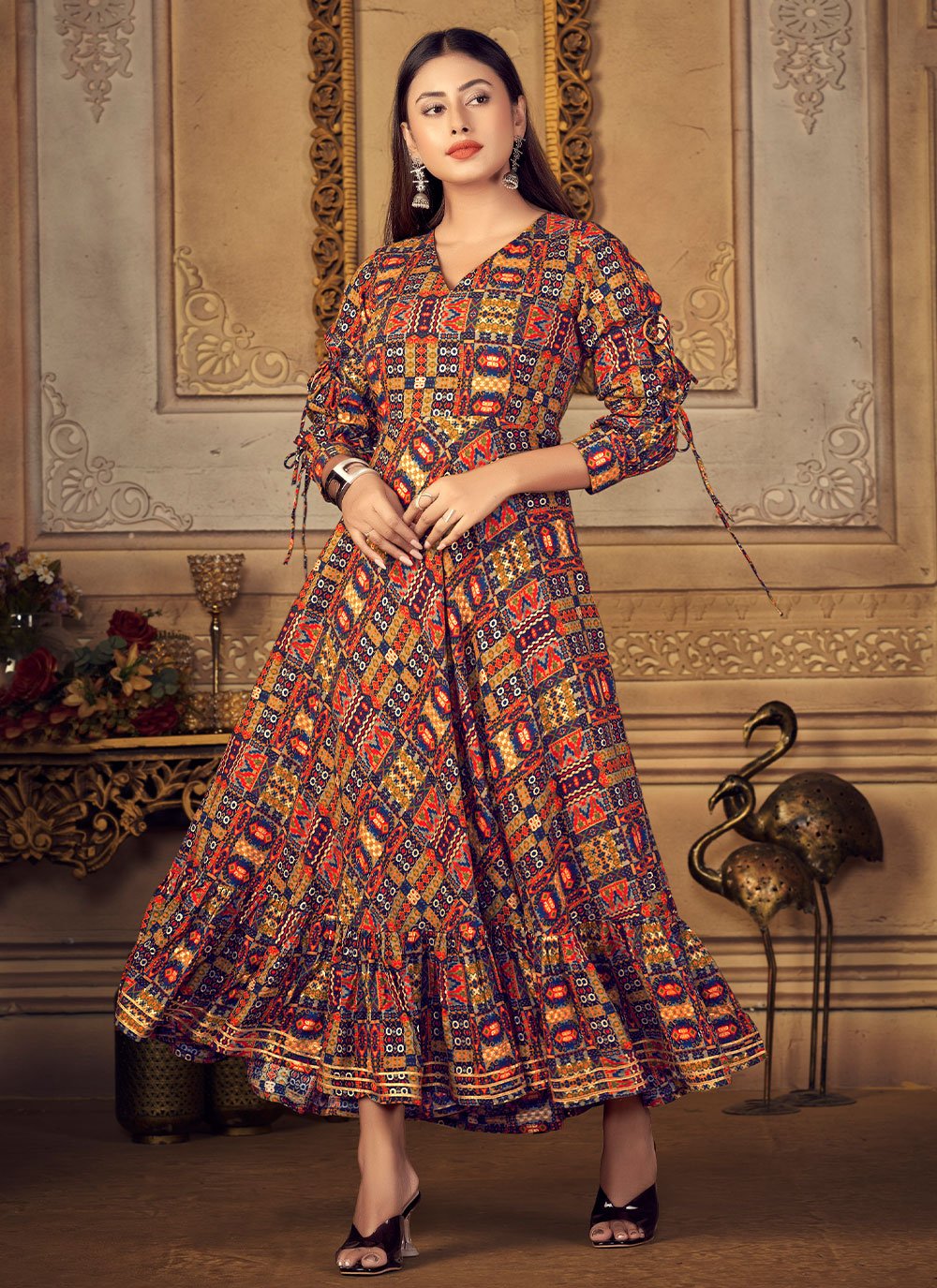This vibrant and meticulously composed portrait captures a young woman in her twenties, of Hispanic descent, standing as the focal point against an ornate, vintage Victorian-style backdrop. She radiates elegance in a flowing, ankle-length v-neck dress adorned with a vivid geometric pattern in rich hues of orange, yellow, and dark blue. Her outfit is complemented by black high heels and an array of jewelry, including a black and white bracelet, several rings, and long, dangling earrings. Her makeup is carefully applied, accentuating her tan skin and red lips. The background features a tan wall with elaborate engraving and framing detail, exuding an air of sophisticated antiquity. Adding to the lavish setting are two metal flamingo sculptures with a copper finish to her right, and a side table holding a chalice, some flowers, and tea lights. The warm brown and soft white tones throughout the décor enhance the overall aesthetic, making this image not just a portrait but a timeless capture intended for a significant event or cherished remembrance.